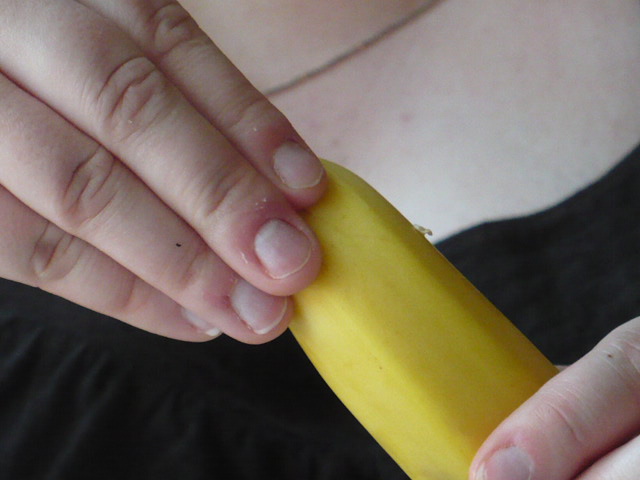In this close-up, landscape-oriented photograph, a young woman with light skin is preparing to peel a yellow banana. At the top of the image, just beneath her neck, part of a thin necklace chain can be seen resting on her chest. She is wearing a black scoop-neck shirt, and a subtle bit of shirring is visible at the neckline. Her right hand, positioned near the banana's stem, is partially obscured but her index, middle, ring, and pinky fingers are visible around the fruit's curvature. Meanwhile, her left hand supports the banana from behind, with the forefinger, part of the middle finger, and a tiny sliver of her thumb visible in the bottom right corner of the frame. The banana is held diagonally between her hands, and it is clear that she is about to peel it, even though the stem remains hidden behind her right hand.